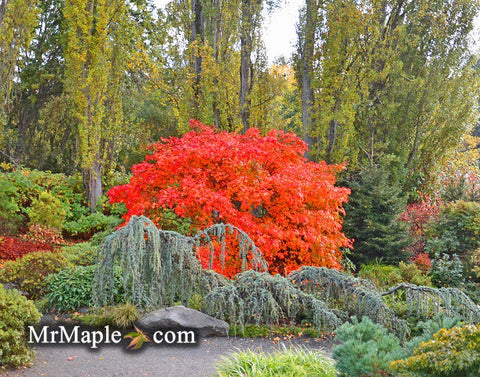This vibrant outdoor scene, likely a park or garden, captures a beautiful blend of foliage and flora. Dominating the center is a stunning, bright orange maple tree, its magnificent foliage immediately drawing the eye. The foreground features a stone walkway leading through an array of low green bushes, some with drooping leaves. On the left side of the image, a mix of green shrubs and a reddish bush adds to the palette of colors. To the right of the maple tree, a baby pine tree stands tall amidst more green and light green bushes, interspersed with a few red flowers. Towering in the background are tall green trees with leaves that extend beyond the frame. The bottom left corner of the image prominently displays the text "MrMaple.com," accompanied by a tree graphic in place of the dot, adding a touch of branding to this picturesque daytime scene.